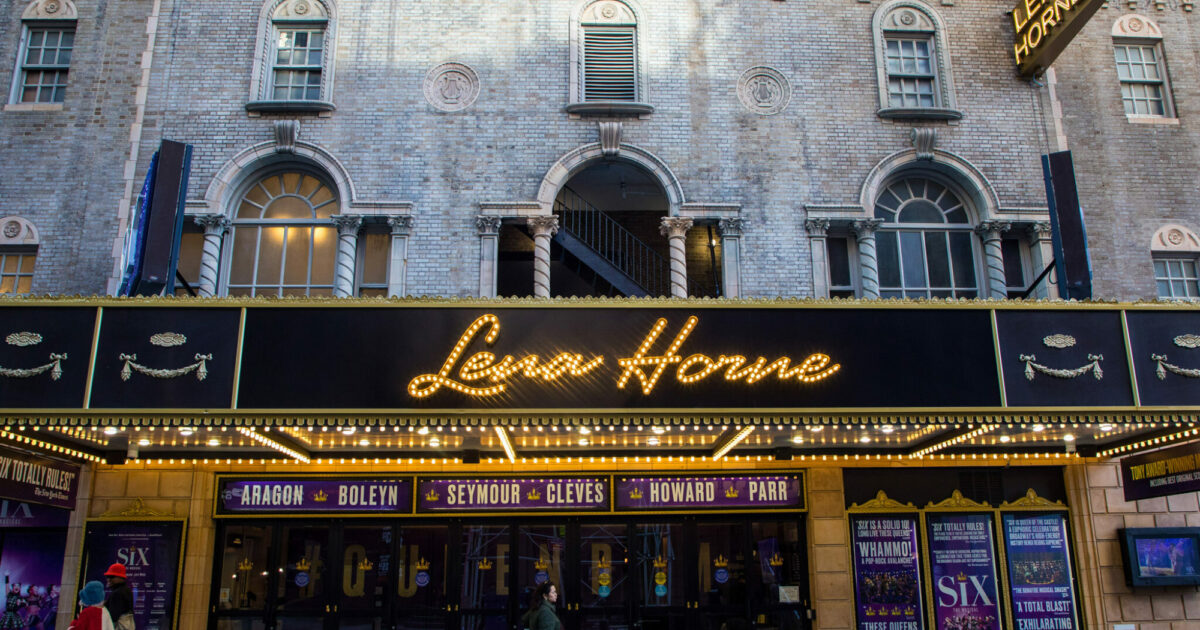The photograph captures the front of an old, brick theater building, distinguished by its grand marquee that proudly displays the name "Lena Horne" in illuminated, cursive letters. This gray, vintage establishment features several large arch windows above the marquee, accompanied by smaller arch windows higher up, suggesting an architectural style from an earlier era. Below the marquee, there is a sequence of smaller purple signs with white writing listing names such as Argonne, Boleyn, Seymour, Cleves, Howard, and Parr, possibly indicating upcoming shows or performers. In front of the theater entrance, with its clearly visible glass doors, a man wearing an orange hat stands out amidst the chilly weather, as indicated by others in jackets and hats. The sidewalk scene includes a few posters promoting various movies and performances, such as one titled "Six," all reinforcing the theater's bustling, local charm.